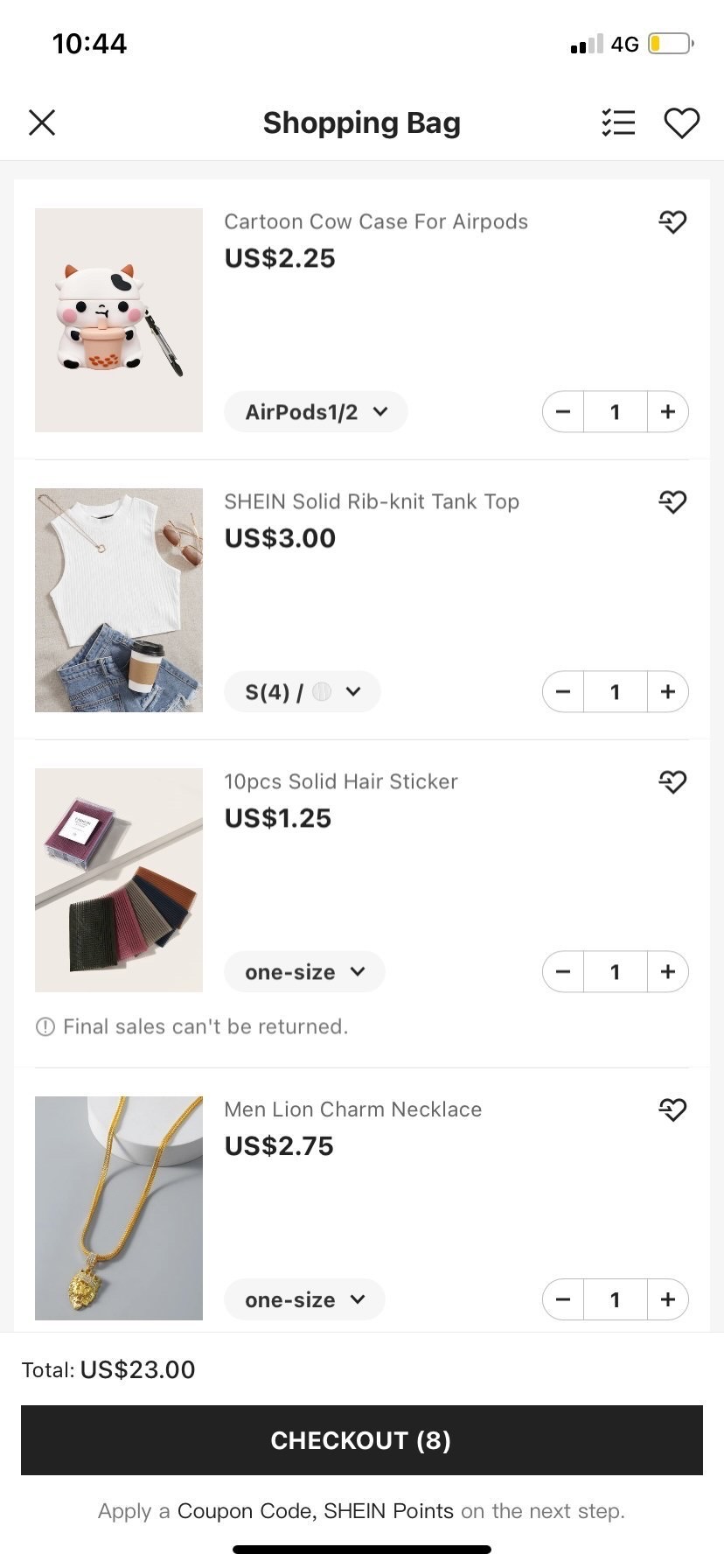The image is a screenshot from a mobile phone capturing an online shopping cart from the Shein app. The entire background is white, providing a clean and simple aesthetic. The cart features a list of items the user intends to purchase, with product images displayed on the left side of the screen. Each product has a detailed description in the center, including the name and price. To the right of each item, there is an adjustable quantity selector, featuring a minus sign on the left and a plus sign on the right, allowing the user to modify the number of items. Each product also has a heart icon in the top corner for users to mark their favorite items.

At the bottom of the screen, there's a black rectangular checkout bar with the numeral '8' prominently displayed, indicating the total number of items in the cart. This bar also includes text that reads, "Apply coupon code, Shein points on the next step."

The list of items in the cart includes a "Cartoon Cow Case" for AirPods priced at $2.25, a "Shein Salad Rib Knit Tank Top" in white, some hair stickers, and a "Men's Lion Charm Necklace." Additionally, there is a small battery icon at the top indicating the phone's charging status.